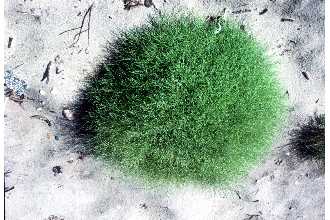The image is a small, almost postcard stamp-sized, top-down photograph displaying a circular, green shrub or possibly a clump of moss. Positioned centrally in the frame, the shrub has a fine, densely packed texture that gives it a puffy, round appearance, reminiscent of a green afro. The background appears to be light-colored, possibly white, grey, or silver sand, and is scattered with twigs, small rocks, and other debris. To the right of the main shrub, there is a smaller, darker clump with a similar texture, which could be a pinecone. The image is not well-focused and is quite pixelated, with the shrub casting a shadow on its left side. There is no text accompanying the image.